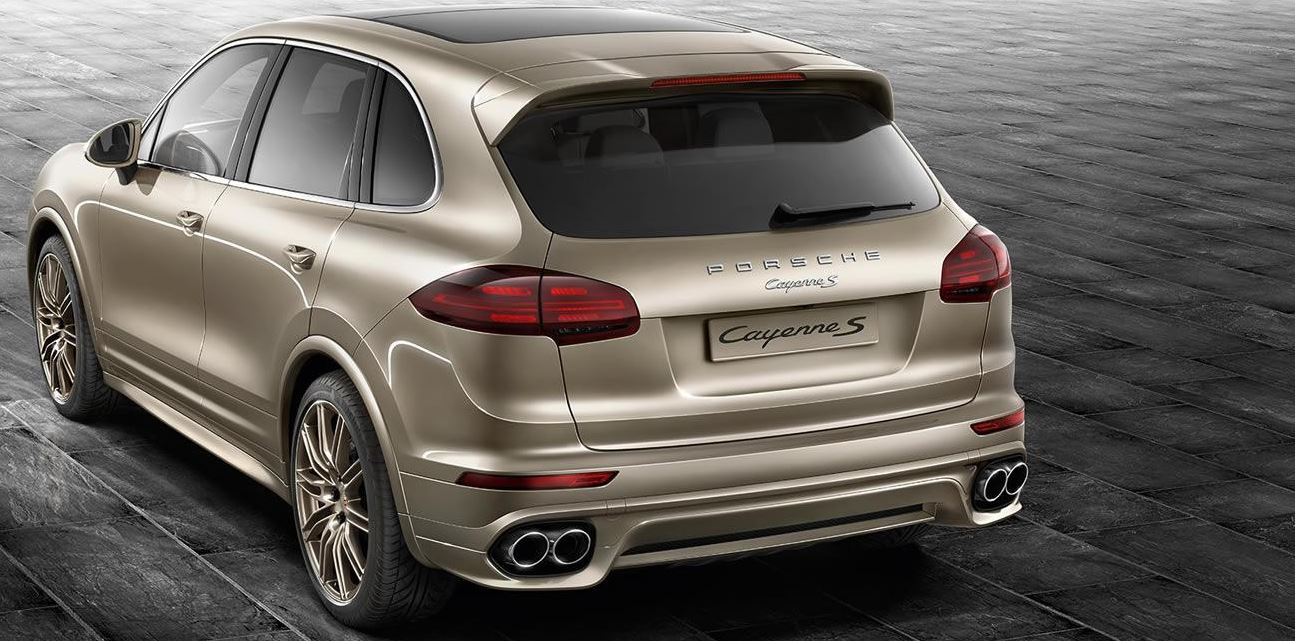This professional, computer-generated advertising photo showcases the rear of a Porsche Cayenne S, depicted in a champagne brown finish that shimmers like gold. The SUV, likely a small crossover, features intricately matched gold rims with black outer wheels. The vehicle's branding is prominently displayed with "Porsche" in text across the trunk just above the rear windshield wiper, and below that, "Cayenne S" is elegantly scripted. A distinctive black sunroof crowns the roof, adding to its luxurious appeal. The background sets a striking contrast with the car, featuring an expansive black marble-like tile patio or paved street, enhancing the elegance of the gold vehicle.